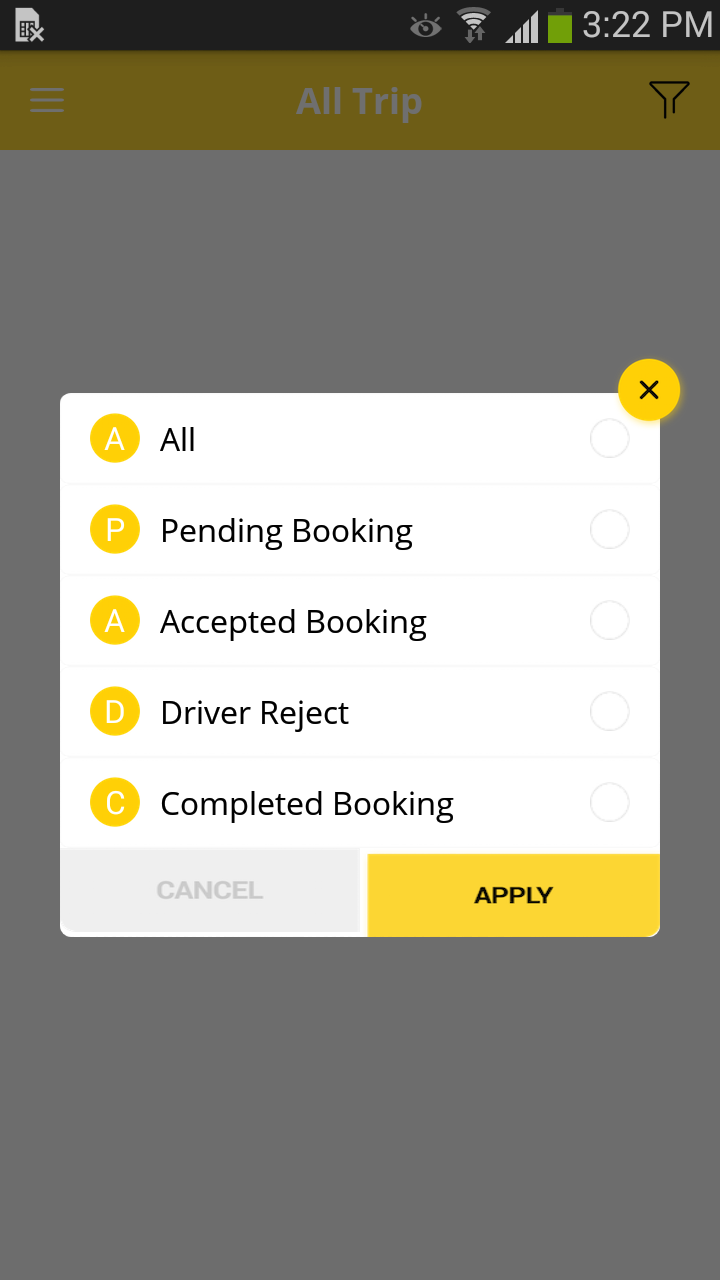In this image, we see a detailed screenshot of a smartphone screen. The screenshot clearly displays the phone's status bar at the top, which includes symbols indicating internet connectivity, signal strength, a fully charged battery, and the current time, which is 3:22 p.m.

The main interface of the screenshot is predominantly yellow and white. A prominent yellow banner at the top of the screen reads "All Trip" against a white background. Below this banner, a central white box is visible, containing options for managing different types of bookings. The options listed are: "All pending booking," "Accepted booking," "Driver reject," and "Completed booking." In the upper right corner of this box is a small 'X' symbol, allowing the user to close the selection menu.

Given these details, it appears that this is a screenshot from a ride-sharing or trip management application. The color scheme is consistently yellow and white, reinforcing the app's branding and user interface design. This app seems to assist users in organizing and managing various trip-related activities, possibly targeting drivers who need to keep track of their accepted, pending, or completed bookings. The user is presumably navigating the app to decide how they want to proceed with their trip management options.